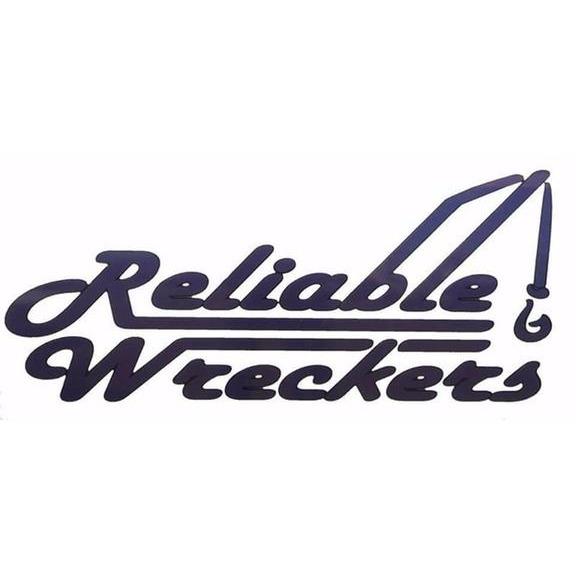The image showcases a logo featuring black text against a white background. The text, written in a bold, easy-to-read font, prominently displays the words "Reliable Wreckers" centered in the design. The word "Reliable" is in italics, with a distinctive feature: the tail of the 'L' extends out to the right, forming a wrecking ball-like object hanging off the end. Additionally, the 'R' from "Reliable" has a unique flourish with its top extending horizontally. The word "Wreckers," in the same font directly below "Reliable," also features an extended horizontal line on the 'W'. The overall design is clean and minimalistic, giving the impression of a professional and potentially industrial or service-oriented brand.